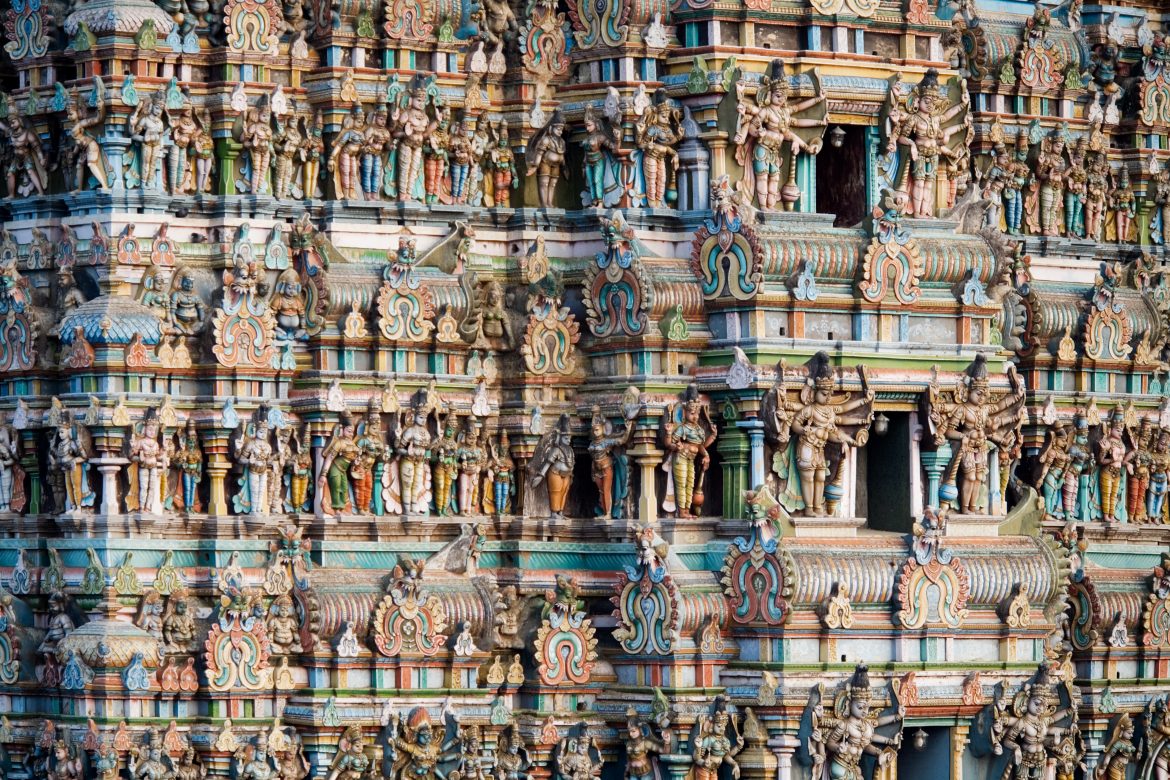This photograph captures an intricate and colorful wall adorned with an array of carved human figures, suggestive of a cultural tableau possibly from Thailand or India. The detailed artistry features multicolored statuettes, predominantly in shades of turquoise, light blue, orange, white, and brown. Central to the composition are two prominent blue columns dividing the wall. To the right of one column are striking figures with multiple arms, specifically six, a motif that repeats with varying attire in statuettes above. These figures evoke imagery associated with Hindu deities, possibly in a temple or shrine setting. The wall itself is embellished with elaborate engravings and varied textures, adding depth and richness to the scene, complemented by accents that resemble shapes like shark teeth. The image showcases entrances interspersed along the grand wall, further emphasizing the ornate and religious aesthetic that's vibrant and captivating.